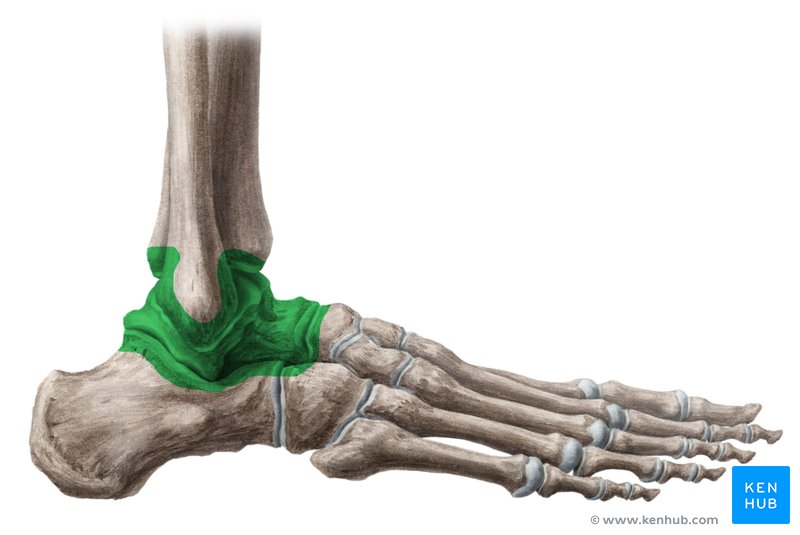This detailed illustration depicts the skeletal structure of a human foot, extending slightly above the ankle joint. The leg is shown descending into the ankle area, which features green shading indicative of cartilage and muscle tissue around the Achilles region. The foot itself is rendered in a bone color with hues of gray and white, highlighting the joints—especially around the elongated toes, which exhibit lighter gray shading. Notably, a small blue square containing the text "Ken" and "hub" is positioned at the bottom right of the toes. The entire image is set against a white backdrop, with the source clearly marked as www.kenhub.com.